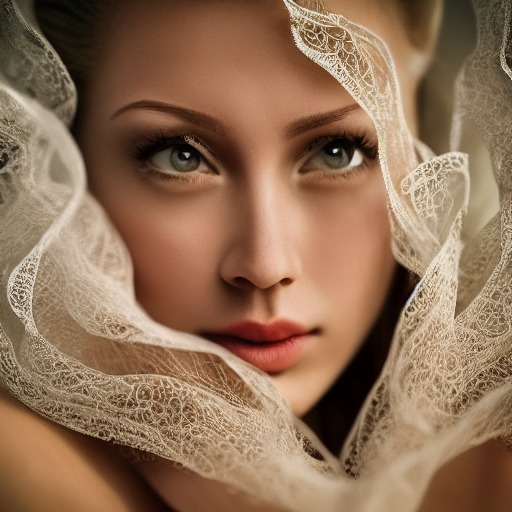This image portrays a woman's face enveloped in a soft, almost dreamlike filter, blurring the line between reality and artistry, suggesting a painted quality. Her eyes, a vibrant green or hazel, are arresting; her right eye appears slightly drifted towards her nose, while her left eye gazes straight ahead. Flowing white fabric delicately frames her face, adding an ethereal touch to the composition. Her eyebrows are meticulously manicured, complementing her striking red lips. Notably, her hair remains hidden, drawing attention solely to her serene and captivating facial features.